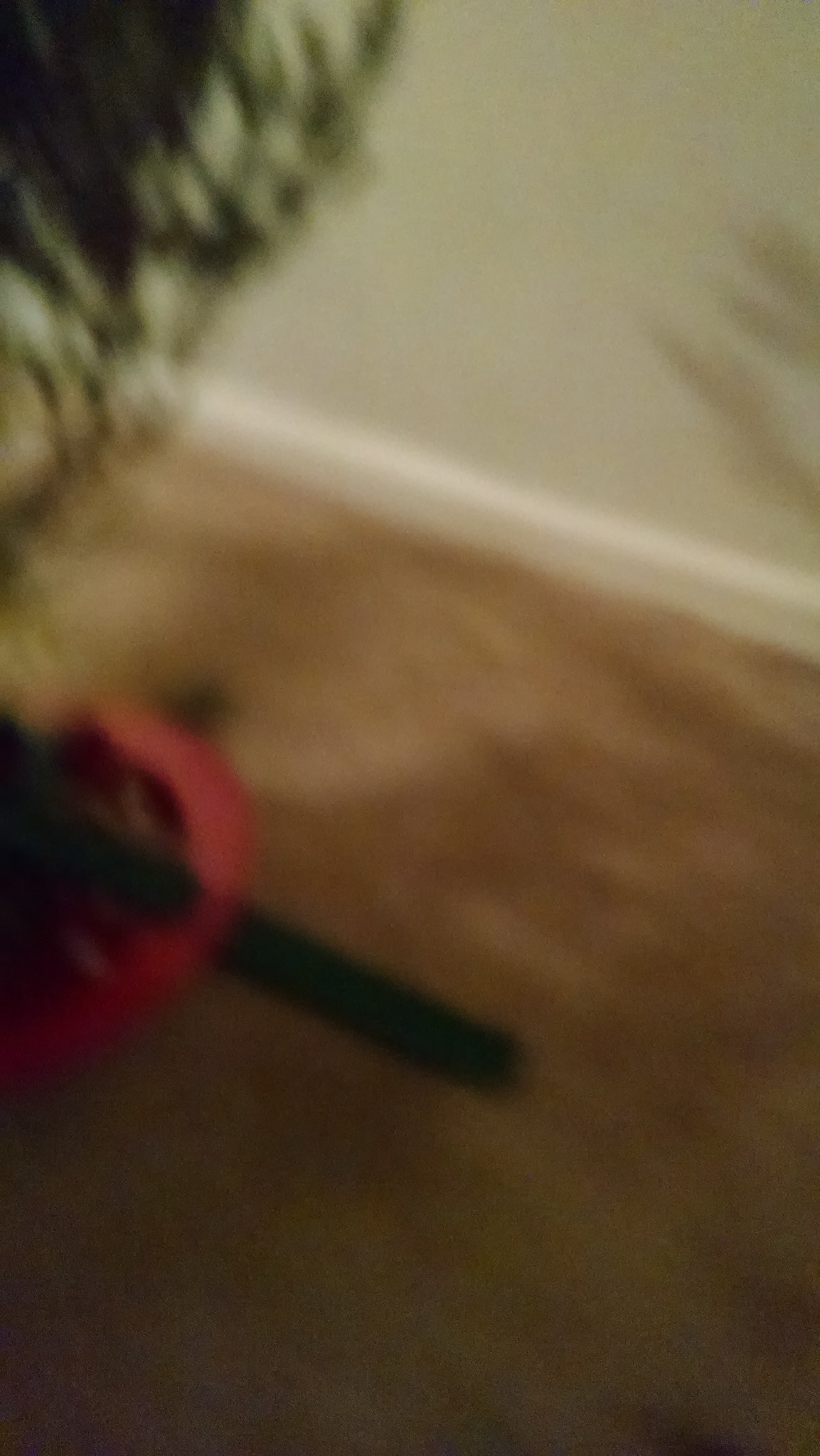This image, though very blurry, captures the base of a Christmas tree stand. The stand features a distinctive red ring that bisects a long green rectangular piece, positioned on a brown carpet. In the upper left corner, a few green branches from the tree can be discerned, contrasting with the off-white wall behind them. Shadows of tree branches fall on the wall to the right. The tree stand itself rests on a carpeted surface that is brown, and a white baseboard trims the wall. There are even hints of green within a very dark, obscured object near the tree stand, suggesting foliage or perhaps a curly element that is difficult to identify due to the image's poor resolution.